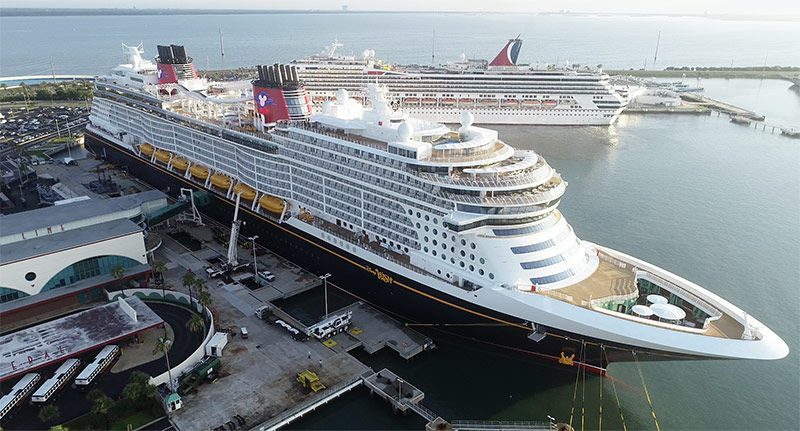The image captures an aerial view of two enormous cruise liners docked side by side. The dominant ship in the foreground is a massive white vessel, rising approximately ten stories high. Its decks are wooden, interspersed with bright yellow lifeboats positioned around the midsection of the ship. This ocean liner features a notable red area at the top near the back with black tubes protruding, adorned with a replica of Mickey Mouse with white ears, indicating a Disney Cruise. At the very top, there is a pool visible. The waters around the ships are a calm, darkish green, extending to the horizon but slightly hazy. The second cruise ship, docked behind the Disney ship, is smaller and bears the insignia of Carnival Cruise Lines. Both ships are facing opposite directions, with the Disney ship orientated to the right and the Carnival ship to the left. The scene also reveals a bit of shoreline to the left, though indistinct due to haziness. Below, near the docks, the entry point for cruise passengers is visible, connected by a staircase leading to a building, with several buses parked in a covered, circular drive area.